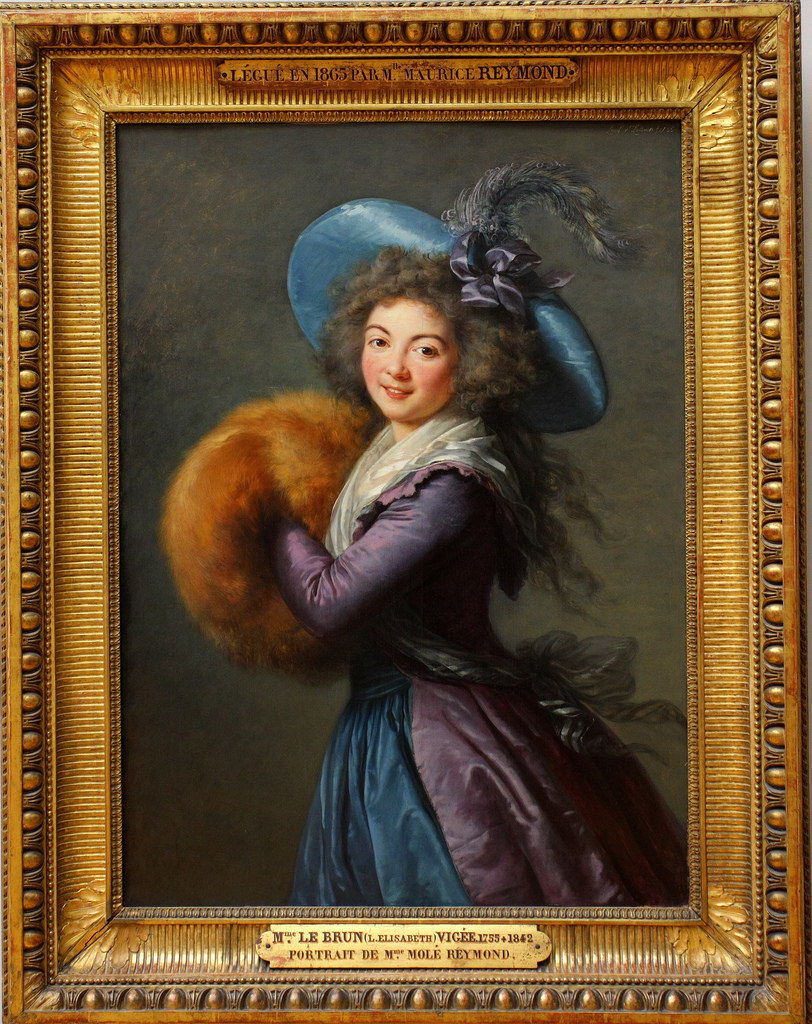A detailed oil painting, framed in an ornate gold or bronze frame, depicts a young woman from the Victorian era. The top of the frame is accented with French inscriptions, reading "Le Gagnon 1865 par M. Maurice Raymond." The painting portrays a young woman with long, curly brown hair, rosy cheeks, and a warm smile. She is adorned in a flowing Victorian-style dress which combines hues of blue and purple, interspersed with white details. The woman is also wearing an elaborate blue hat decorated with a long feather and a purple ribbon. In her hands, she carries soft, orange pom-poms or a fur muff to keep warm. Below the painting, an inscription on the frame reads "LeBrun Elizabeth" and further details include "Le Brun Vigres, 1785-1842. Portrait d'Aime-Mont-Raymond," indicating the artist and possibly the name of the muse.